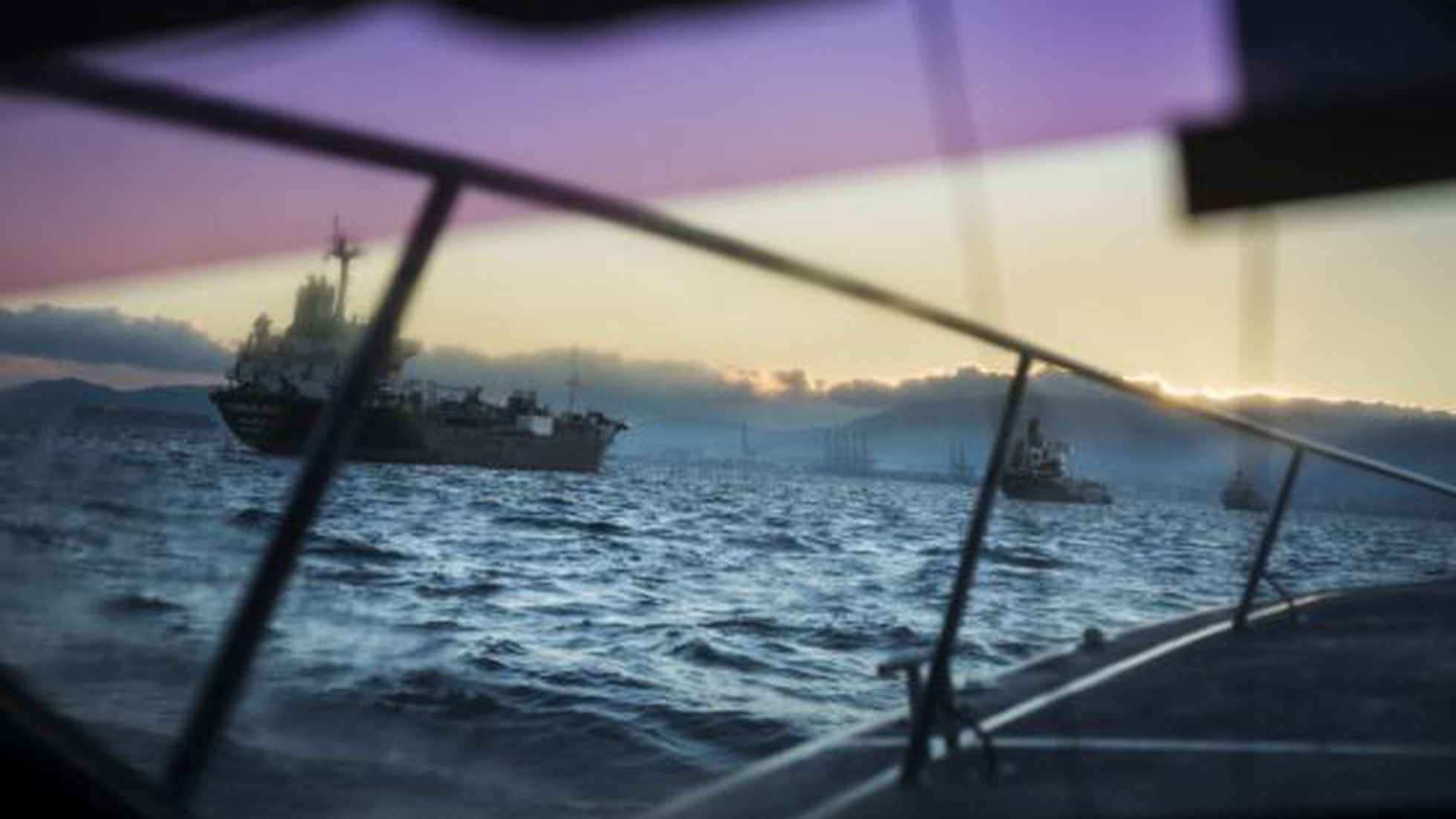This horizontal photograph captures a tranquil harbor scene observed from the deck of a boat. The vantage point is from behind a silver railing, complete with cleats for securing ropes, suggesting the deck's proximity to the viewer. In the midground, three gray boats, possibly military or tugboats, float on dark, almost black water, moving left in a neat row. The water stretches toward a horizon that is partly cloudy, suggesting a serene morning or late afternoon ambiance. The sky above features a bank of clouds, softened by the muted light, giving a sense of either sunrise or sunset. In the top right of the image, partially obscured elements, including a purple rectangle and a yellow patch, hint at possible obstructions on the camera lens or artifacts from a sun visor. The overall composition immerses the viewer in the quiet, contemplative atmosphere of the harbor, as seen through the eyes of someone standing on the boat deck.